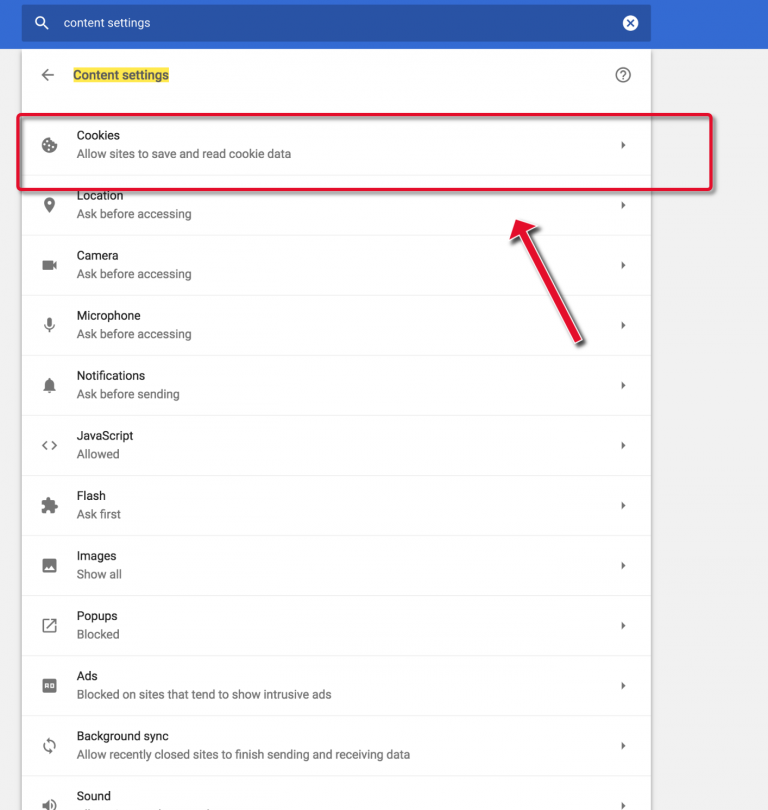This is a detailed image captured from someone's computer screen displaying the "Content Settings" section of a web browser. At the top of the image, there's a blue rectangular bar, which contains a smaller navy rectangle featuring the text "Content Settings" alongside a magnifying glass icon. 

Directly below, the phrase "Content Settings" is prominently highlighted with yellow and an arrow pointing to the left. Below this highlighted section, there is a specific area labeled "Cookies," identifiable by an image of a cookie with a bite taken out of it. Next to the image, the option "Allow sites to save and read cookie data" is displayed.

An additional emphasis is created around the "Cookies" section by a red rectangle, drawn to encase it, complemented by a red arrow pointing towards this boxed area. 

As the eye travels further down the image, it encounters sections dedicated to managing various web permissions and settings including Location, Camera, Microphone, Notifications, JavaScript, Flash, Images, Pop-ups, Ads, Background Sync, and Sound. Each of these sections is neatly arranged, indicating comprehensive control options for the user’s browsing experience.